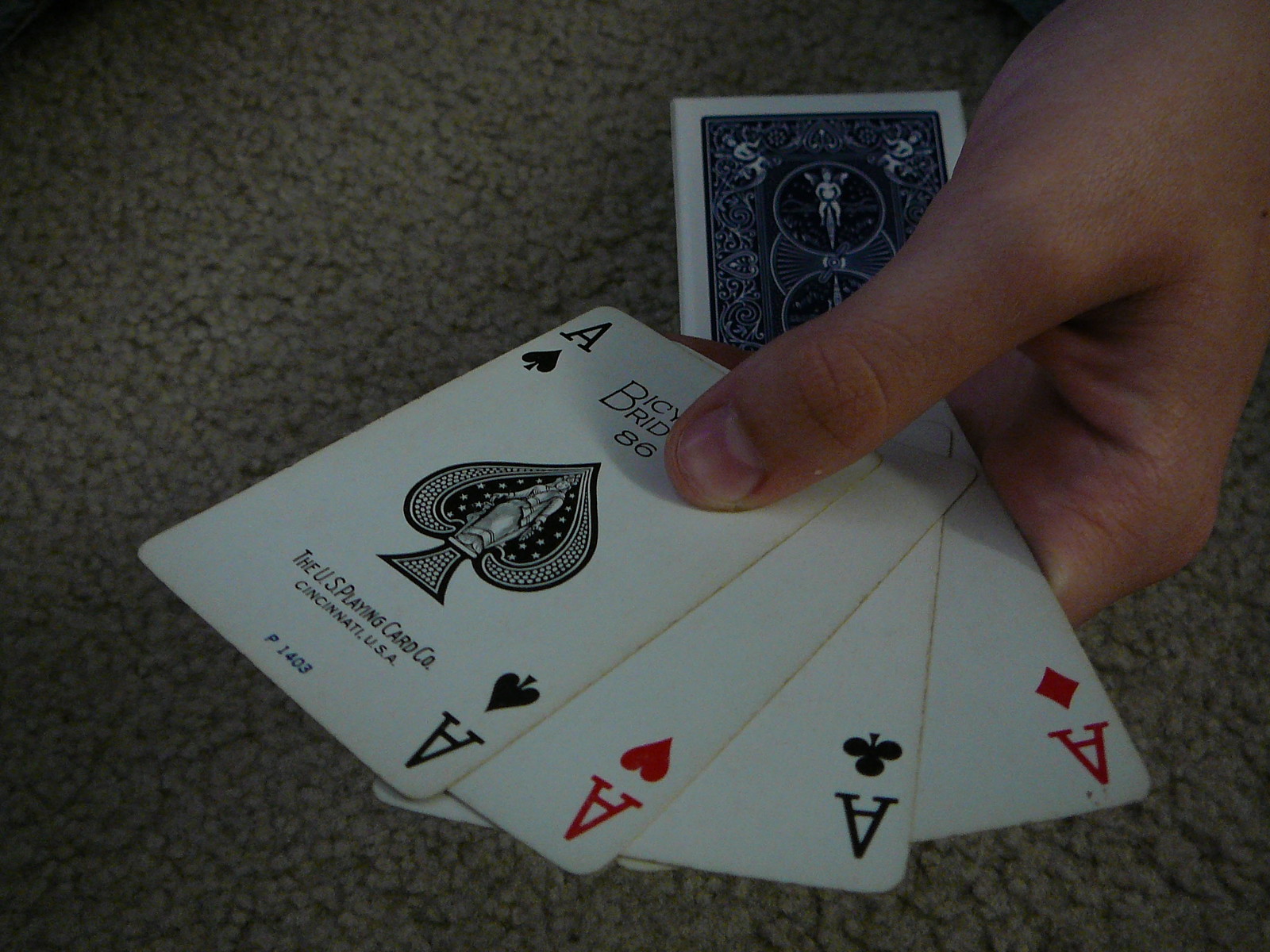A digital indoor photo captures a close-up view of a hand holding four aces of playing cards against a background of a grayish or colored carpet. The lighting creates a gradient effect, making the upper right portion of the image brighter and the upper left and bottom parts darker. The Caucasian hand, descending from the upper part of the image, grips the cards with the thumb positioned on the top left card. The cards are fanned out, displaying the faces in a sequence from right to left. They are upside down, starting with the Ace of Diamonds on the right, followed by the Ace of Spades, the Ace of Hearts, and then another Ace of Spades as the top card.

The top card features intricate detailing, with "BICYCLE" printed at the top and "86" underneath it. The card showcases an ornate black and white spade design in the center, with "The U.S. Playing Card Co." inscribed below, followed by "Cincinnati, USA" on the next line, and "P1403" at the bottom. Behind the hand, the rest of the deck lies face down, with a white border and an elaborate blue design filled with white stenciling.